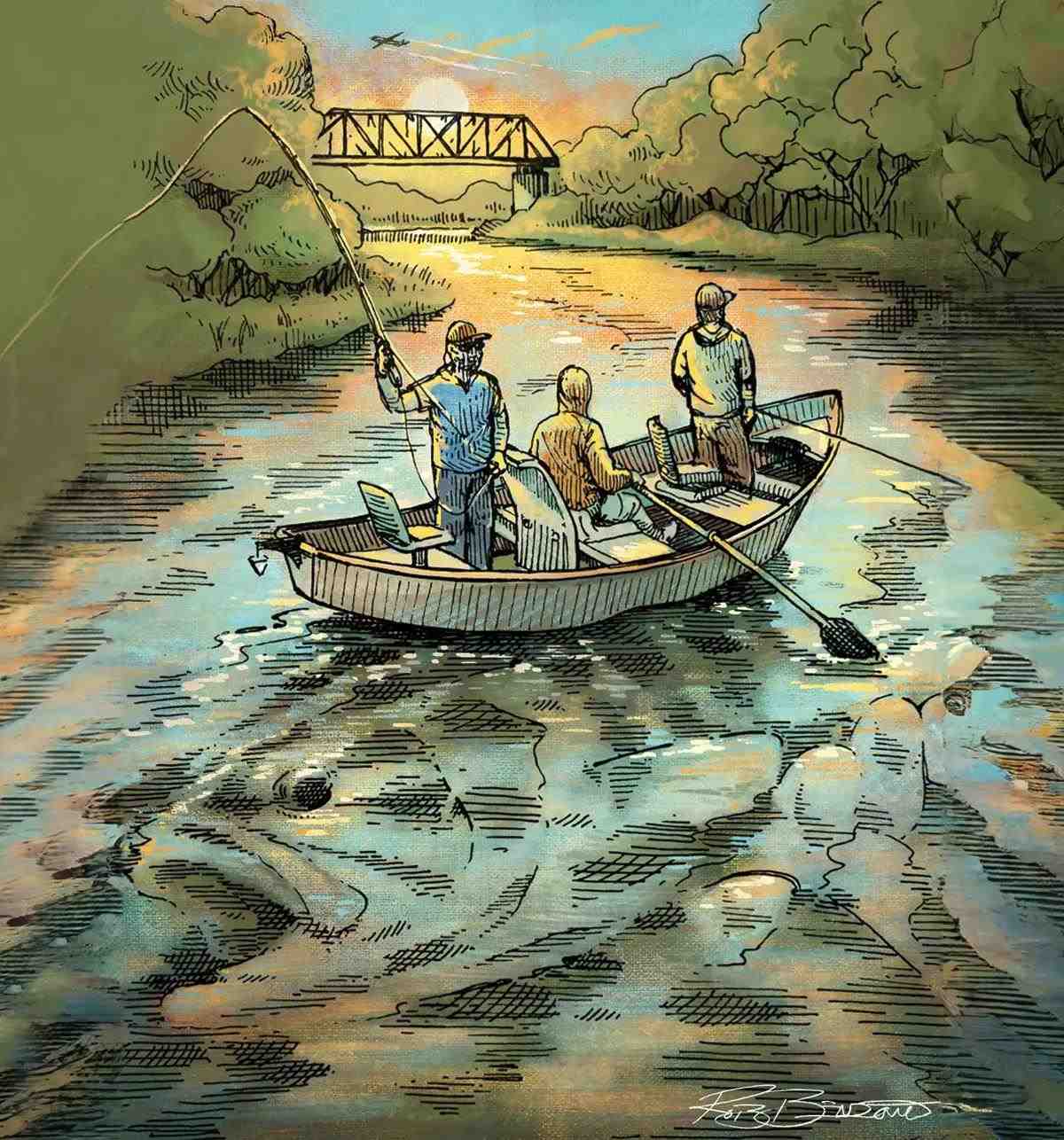The illustration shows a small paddle boat with three people engaged in fishing on a river. The boat is centered in the image, and the detailed cross-hatching brings a richness to the black line work. One person, located at the front of the boat, is casting a fishing line into the water, while the middle person is seated and paddling. The third individual, standing towards the upper part of the boat, appears to be overseeing the fishing efforts. Below the surface of the water, defined by intricate black lines, is the enormous outline of a sea bass with its mouth wide open, measuring almost twice the size of the boat, unbeknownst to the fishing trio. The background features lush green trees and foliage on either side of the river, a cross bridge, and an airplane flying overhead. The sky shows a setting sun casting an orange reflection on the water, enhancing the painting's serene yet suspenseful atmosphere.